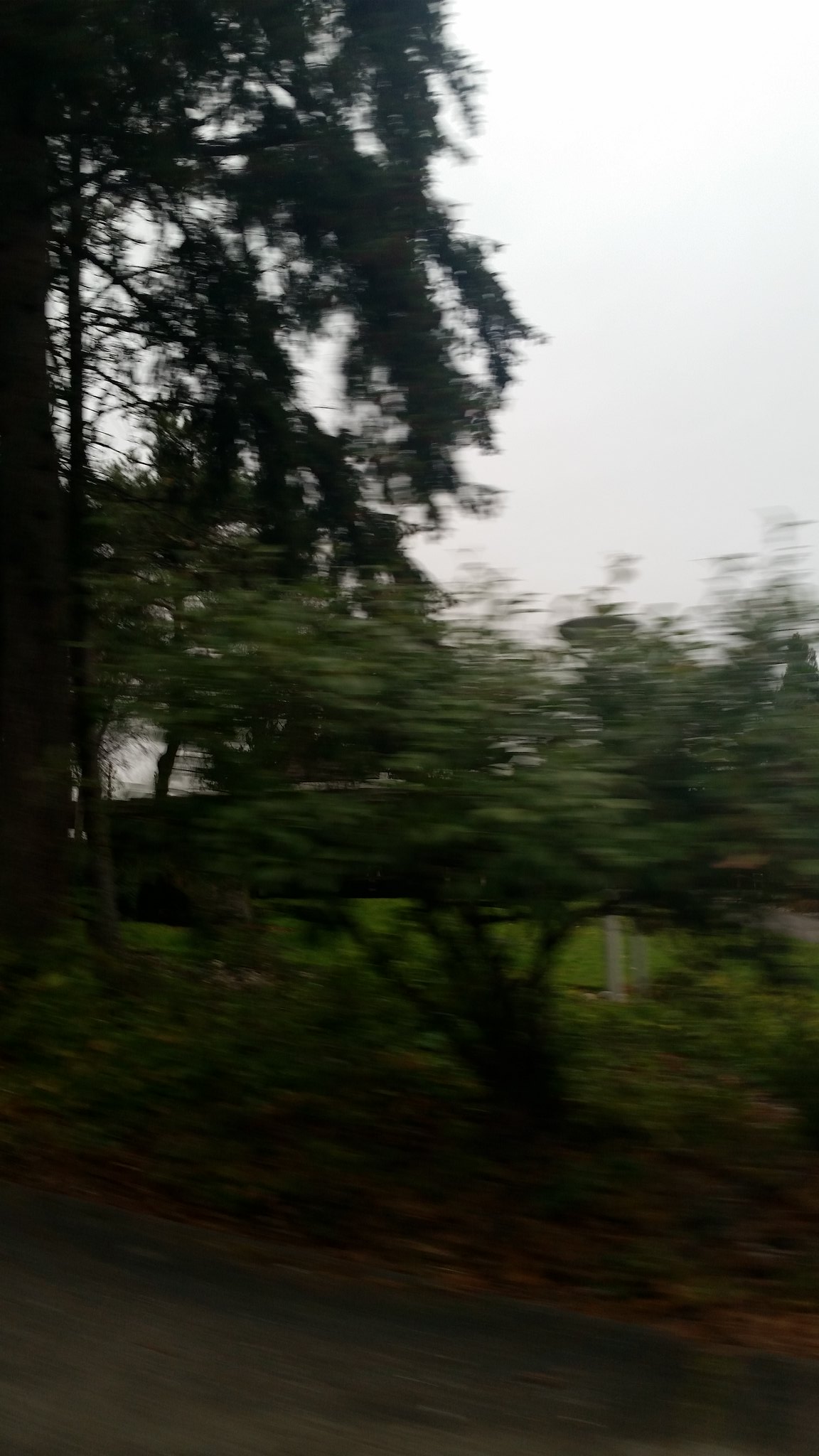This outdoor photograph is blurred and showcases a scene possibly at a golf course, nature park, or wooded area. Dominating the top left of the photo, a tall tree, likely an evergreen although hard to confirm due to the low light and blur, extends nearly the full height of the image. To the middle of the frame, some shorter trees stand at about half the height of their taller counterparts. Lower vegetation and small trees scatter the middle portion, though they are difficult to distinguish clearly. The sky throughout the upper right part of the photo has an overcast, white appearance, suggesting either dusk or a cloudy day.

The bottom part of the photograph reveals a dark gray, possibly cobblestone, road with visible rocks and unevenness, creating a stark, black foreground. This heavily shaded area might imply the picture was taken from within a shaded or darkened space, like a car. Additionally, behind the tree line, a fence with possible chicken wire can be faintly seen, adding to the rustic, natural atmosphere of the scene.